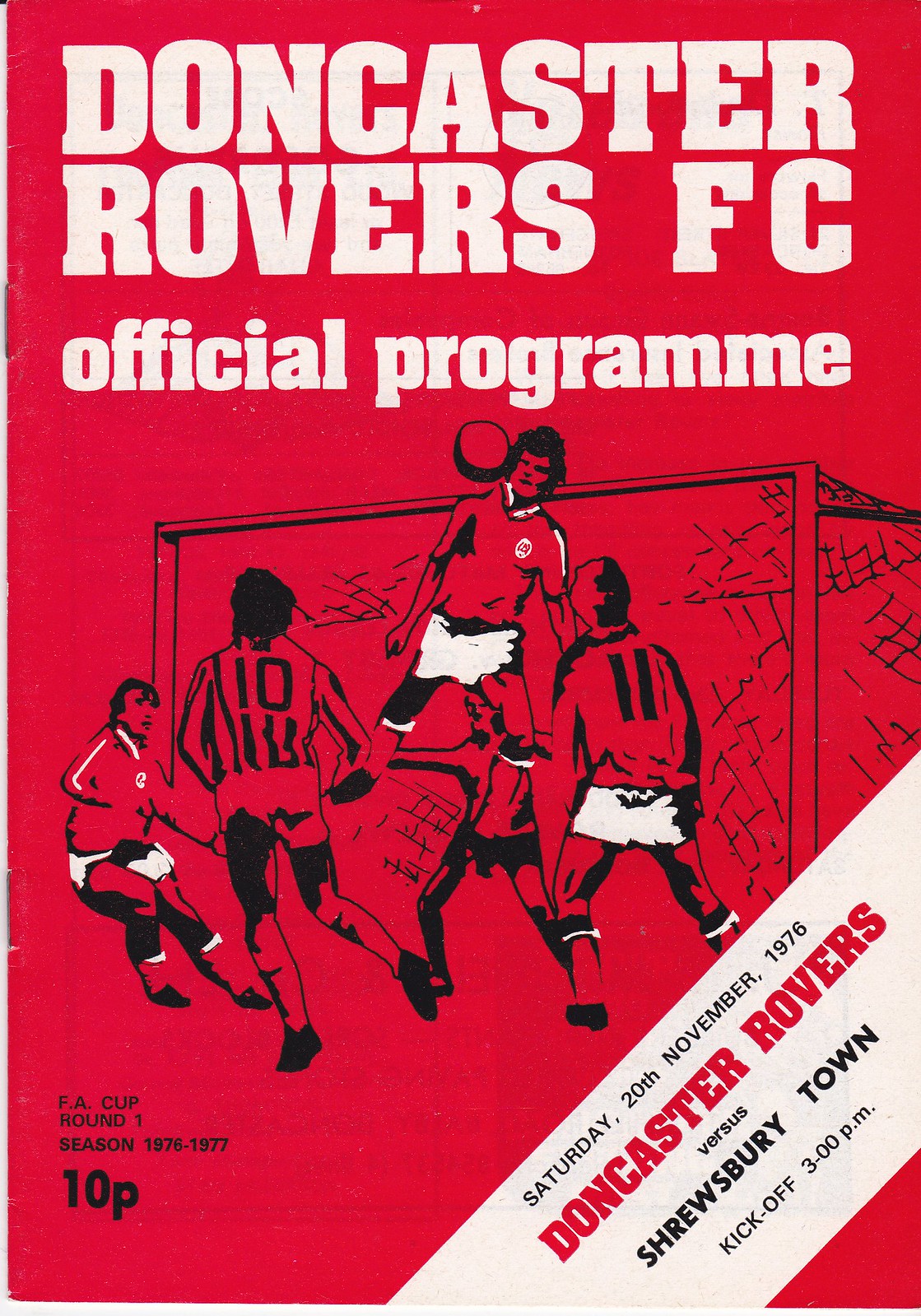The image is a vintage program cover for the Doncaster Rovers Football Club, displaying a rich red background with prominent white text. At the top, the title reads "Doncaster Rovers FC Official Program." Below this, an intricate black ink drawing depicts an intense soccer scene: a goalie with outstretched arms is attempting a save while a teammate in white shorts jumps to block the ball with his chest. Surrounding them are three other players; one seems to be mid-run, and two are looking towards the leaping player, their backs to the viewer, wearing numbers 10 and 11 respectively. The lower right corner features a white diagonal banner that provides event details: "Saturday, 20th November 1976, Doncaster Rovers vs Shrewsbury Town, kickoff at 3 p.m." Additionally, the bottom left corner notes the price, "10 pence," and specifies the "Season 1976-1977." This evocative poster captures a moment in football history with detailed visual and textual elements.